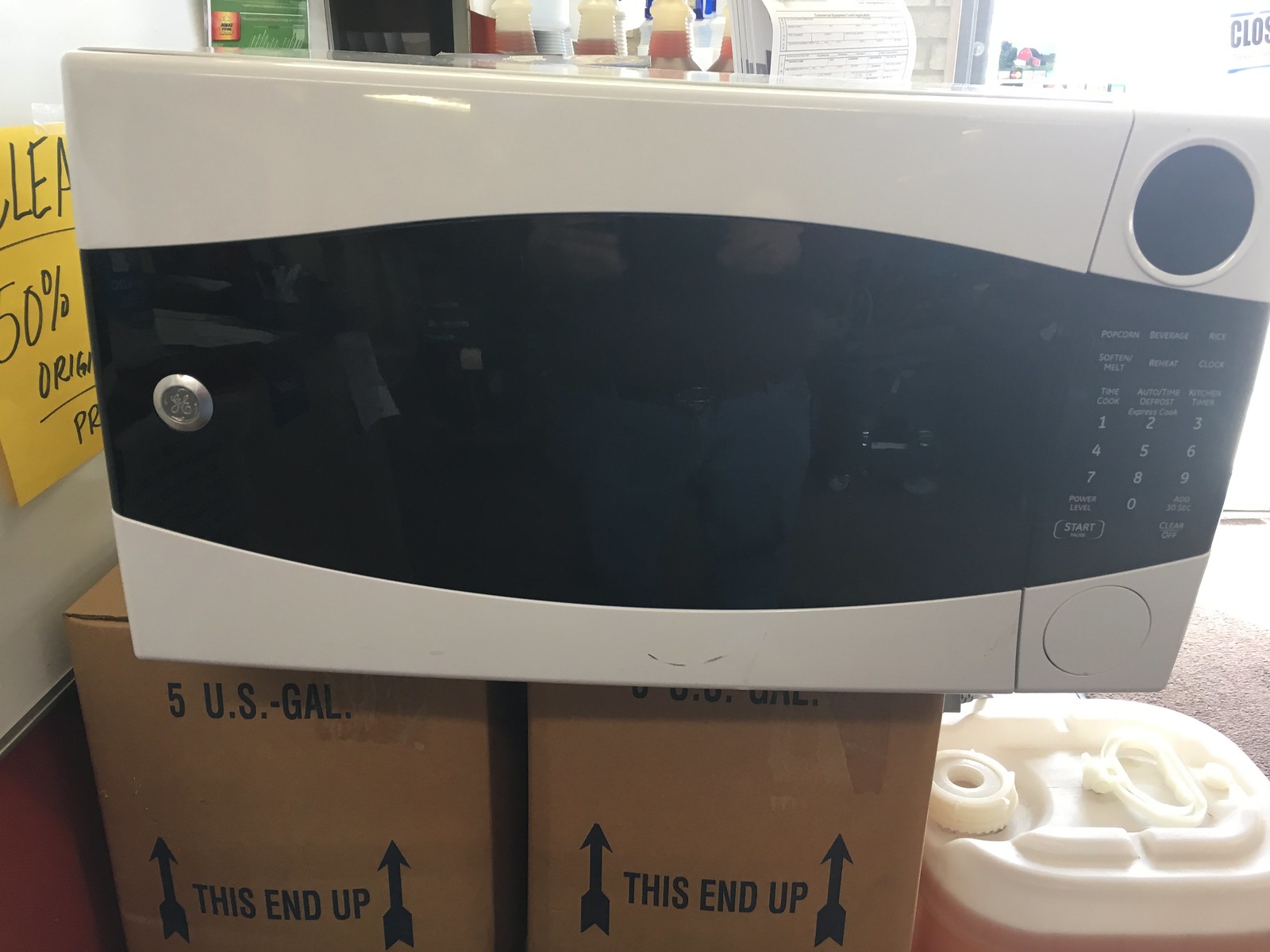This image depicts a white microwave oven with a black control panel and screen, prominently displaying the GE logo on a metallic button. The microwave, which has a range of functions such as numbers 1-9, start, clear, power level, and preset buttons for popcorn, beverages, and rice, is shown sitting on two cardboard boxes. These boxes are marked with "5 US gallon" and "this end up" indicators. Behind it, there is a yellow sign that indicates a 50% discount off the original price, which suggests the microwave is on sale in a store. The background features additional products, including bottles of brown liquid and cleaning supplies, likely in a liquidation shop. A store window is also visible, reflecting the person taking the picture, who is dressed in light wash jeans, a black belt, and a tucked-in long-sleeve shirt. Below the microwave, there appears to be some styrofoam packing material. The scene captures a bright, indoor retail environment with various items on sale.